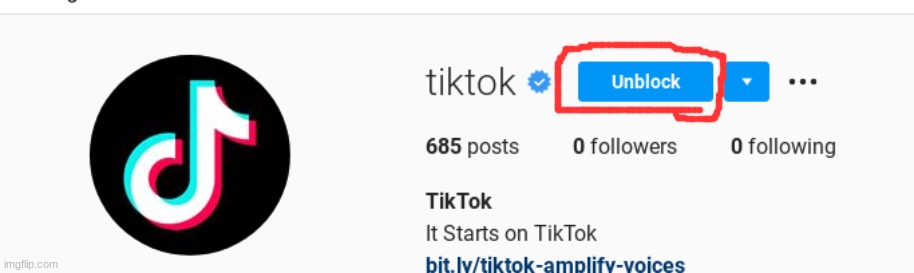This image, related to the TikTok app, features various graphical elements arranged on a light gray background. In the bottom-left corner, in very small print, the source "imgflip.com" is noted.

Dominating the left side of the image is a large black circle with the TikTok logo prominently displayed. To the right of the logo, the text "TikTok" is written. Adjacent to this setup is a blue circle, resembling the rays of the sun, with a white check mark at its center.

Next to the blue circle is a blue rectangle outlined with a thick, hand-drawn red border. Inside this rectangle, the word "unblocked" is displayed in white text. To the right of this rectangle, there is a blue square featuring a small white arrow pointing downwards. Proceeding further, three black dots are aligned horizontally across the page.

Below these graphical elements, the text "685 posts, zero followers, zero following" is displayed, followed by the word "TikTok." The subsequent line reads "it starts on TikTok," and the image concludes with a URL in blue text: "bit.ly/TikTok-amplify-voices."

There are no additional images, text, or photos present on this page.